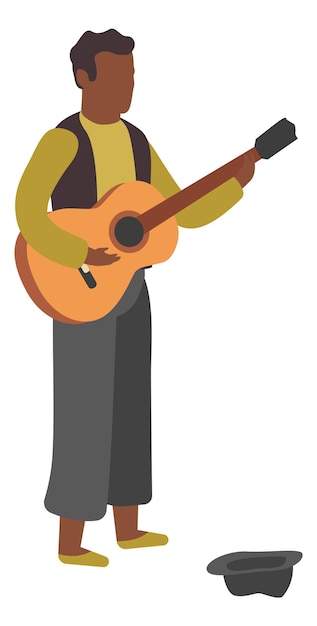This detailed illustration in portrait orientation features a street musician drawn in a cartoon style. He has dark skin, dark brown hair, and no facial features. The musician is depicted holding an acoustic guitar, which has an orange body, a brown fretboard, and black tuning pegs. He wears a black vest over a yellow long-sleeved shirt, paired with dark or gray pants, and yellow slippers. The image lacks a background, suggesting he is standing on a street, playing and possibly singing. An upside-down hat placed in front of him is meant for passersby to toss money into as a donation for his performance. The body of the musician is characterized by simple shapes in solid color segments, reflecting the cartoonish style of the illustration.